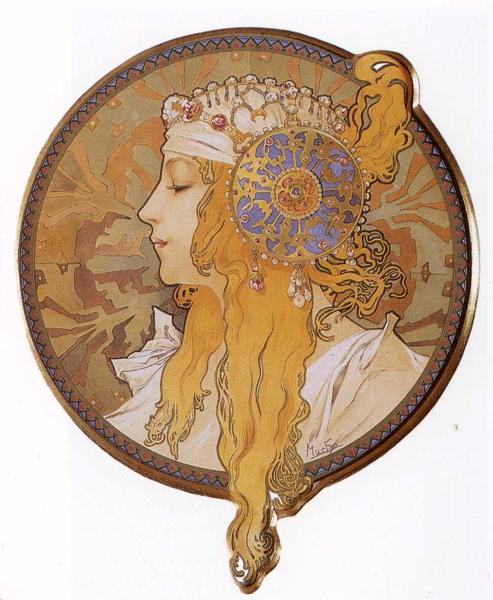The image features a round, gold-colored medallion set against a white background. The medallion has a vintage appearance, reminiscent of a style from the late 1800s to early 1900s. It is bordered by small triangular spikes and contains an abstract background filled with shades of yellow, orange, and brown on a tan backdrop. At the center of the medallion is a side profile of a Caucasian European woman with long, strawberry blonde hair that extends beyond the circular border. She is adorned with a white, bejeweled scarf, which includes gold and red gems, and a large circular blue and gold barrette with hanging jewels. A feather, matching the color of her hair, rises from the barrette. Her attire consists of a frilly white top or dress, revealing only her head and part of her chest. The woman’s eyes are closed, adding a serene quality to her depiction.